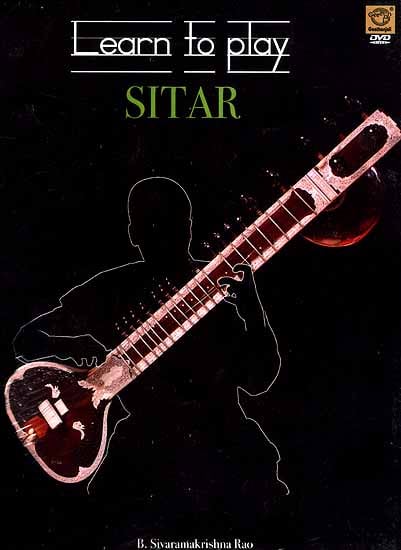This image is a detailed black DVD cover for an instructional video on learning to play the sitar. The cover prominently features the text "Learn to Play" in white, capital letters at the top, flanked by white horizontal lines reminiscent of lined paper used by beginners. Beneath this, "Sitar" is boldly displayed in green capital letters (S-I-T-A-R). The backdrop is solid black, enhancing the design elements. 

There is a striking visual of a person outlined in white, set against the black background, giving a shadow-like effect without any facial features. This figure appears to be playing a sitar, which is depicted with a dramatically long neck. The sitar itself is visually captivating, with a red, glowing effect highlighting it against the dark background. The body of the sitar is comparatively smaller, creating an exaggerated contrast.

On the top right, there is a barely readable emblem with the words "DVD," indicating the format of the instructional content. The bottom of the cover bears additional text that seems to read "Be Silverneck Rishna Ras," though the full message is unclear.

Overall, the cover combines striking visuals and clear typography to effectively advertise the instructional DVD for learning to play the sitar.